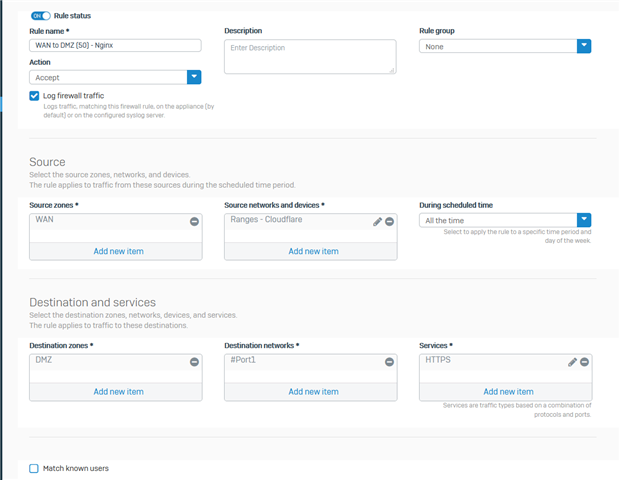This image appears to be a screenshot of a configuration page for setting up Wi-Fi or a home network. 

The layout includes an oval-shaped indicator, and on the right side of the oval, there is a white dot. Within the blue part of the oval, the text "On" is displayed in white font. Below this section, you find labeled areas for rule configuration. The "Rule Status" label precedes a field for "Rule Name" marked with an asterisk, indicating it is a required field. The current rule name is "WAN to DMZ 50," displayed in a rectangular text box.

At the top center, there is another rectangle labeled "Description," with a text box prompting "Enter description," where users can input further details.

The page features a "Rule Group" dropdown menu, currently set to "None," and another dropdown menu labeled "Action" displaying the word "Accept." Nearby, a blue check mark next to the text "Log Firewall Traffic" indicates that logging is enabled.

The "Source" section invites users to "Select Source Zones, Network, and Devices." Below this instruction, two boxes are displayed. The "Source Zones" box currently contains "WAN," and the "Source Network Devices" box lists "Ranges Cloudfair," with an option for users to add new items in both categories. 

The text "Destination and Services" appears next, where the "DMZ" is highlighted, accompanied by "#Port 1," and "HTTPS" is also listed.

This page is likely used for defining network rules, including specifying sources, destinations, actions, and logging preferences.